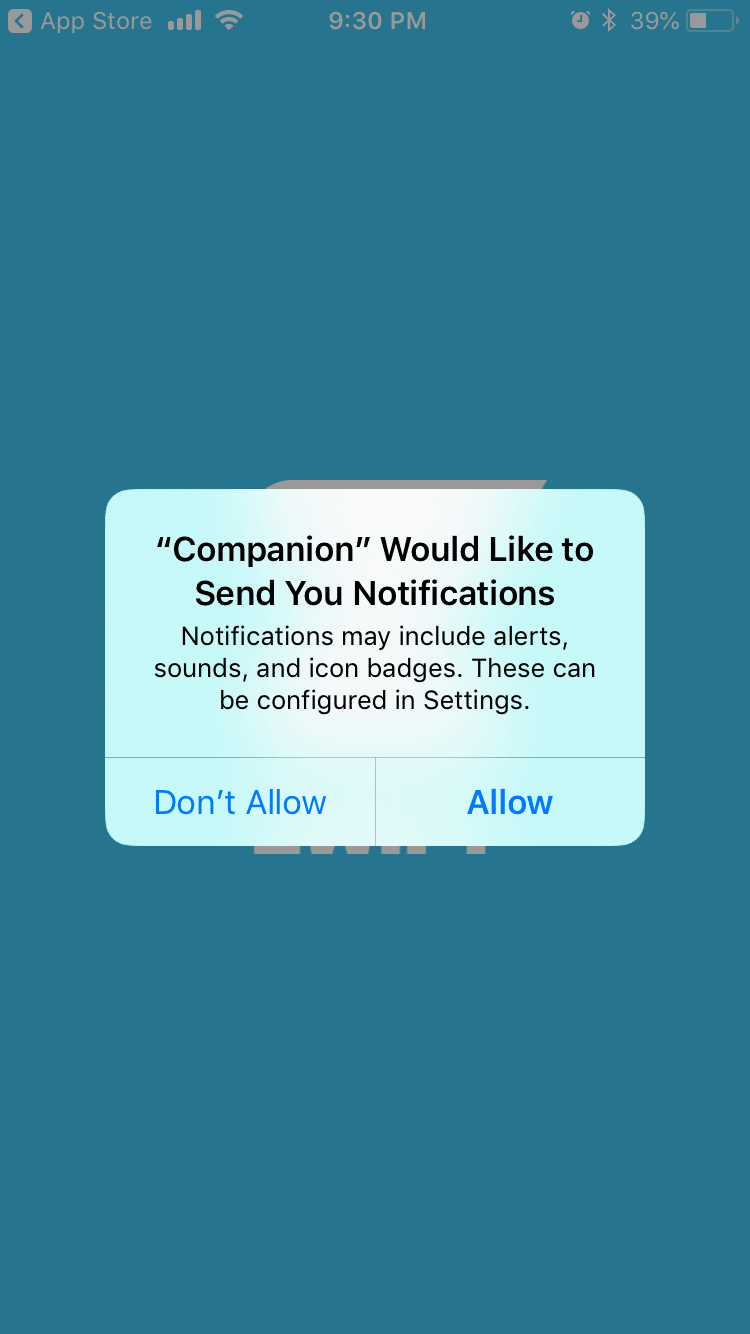The image displays a pop-up dialog from an app called Companion, requesting permission to send notifications. The dialog box outlines that notifications may include alerts, sounds, and icon badges, and mentions that these settings can be configured later. The text within the dialog is black, with two options at the bottom: "Allow," which is in bold blue text, and "Don't Allow," in regular blue text. The rest of the screen is grayed out to focus attention on the pop-up. The background of the dialog is blurred, and appears to be part of the Companion app interface, which is predominantly in a solid bluish or aqua teal color, suggesting the user is opening the app for the first time. At the top of the screen, there is a back button labeled to return to the App Store. Additional details on the device include a 39% battery life and an alarm set for 10:30 PM. The name ‘Companion’ implies functionalities related to home automation or location tracking.